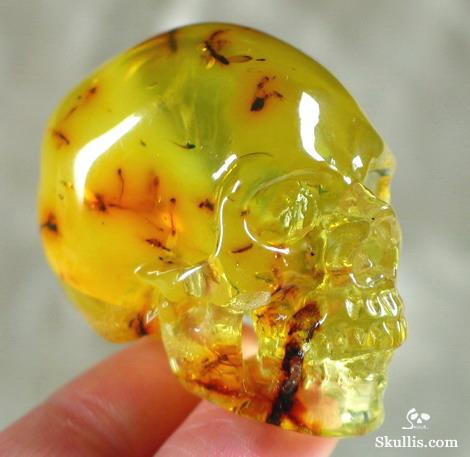The image showcases a close-up, color photograph of a small, yellow skull that appears to be made from a translucent, shiny material, possibly hard plastic or a gemstone like amber. The skull exhibits amber and reddish-orange tints, with brown spots that resemble plant matter or insect fragments trapped within the material. The reflective, jelly-like surface of the skull catches and reflects light, adding to its glossy appearance. The skull is held delicately between the index and middle fingertips of a Caucasian hand, emphasizing its miniature size. In the bottom right corner, there is a watermark that reads "Skullis.com" accompanied by an image of a skull.